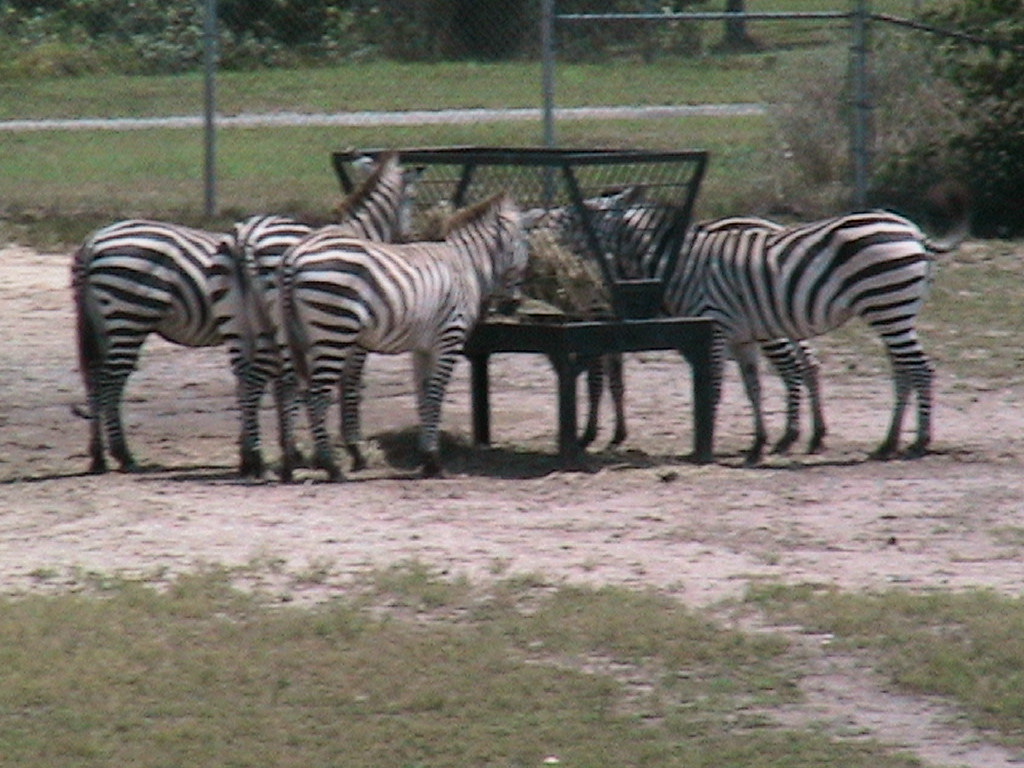The image depicts a group of zebras, ranging from four to five in count, inside an enclosed area likely within a zoo or animal viewing facility. The zebras, characterized by their distinctive black and white stripes, are standing on a dry, worn-out ground with some patches of shrubbery and sand, devoid of lush grass. They are gathered around a trapezoid-shaped metal container, which appears to be part of a feeding structure, likely filled with hay. The photograph, seemingly taken from a distance with an older camera, shows the zebras facing away from the viewer, obscuring their faces. In the background, outside the fenced area, patches of grass and a few trees are visible, contrasting with the barren ground inside the enclosure.